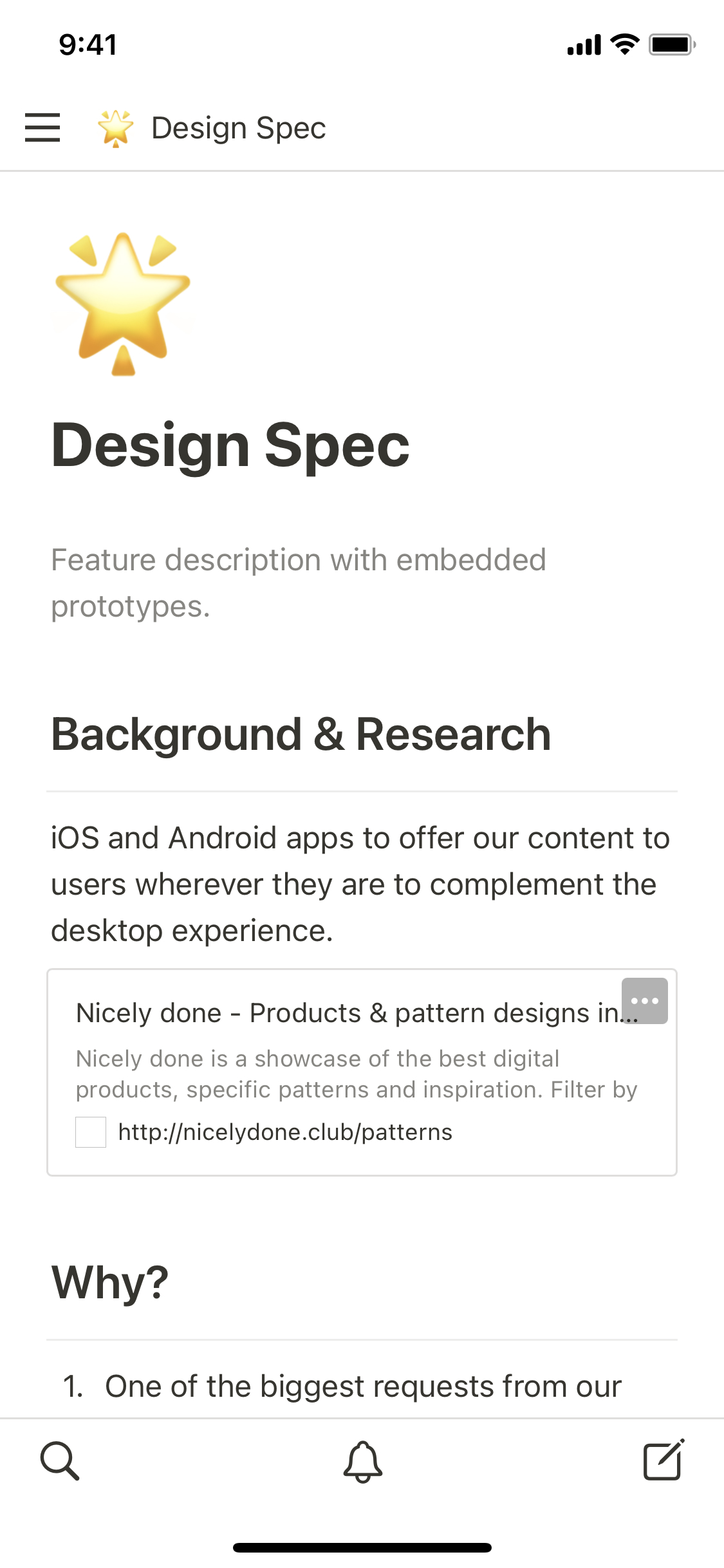Screenshot 941 displays several important UI elements: 

- The top left and right corners feature icons for service bars, Wi-Fi connectivity, and battery life, ensuring users can monitor device status.
- Below these icons, the phrase "Design Spec" is prominently displayed.
  
The main content of the screenshot showcases a detailed description of a "Design Spec" feature, including:
- Embedded prototypes
- Background research
- iOS and Android apps to deliver content universally, enhancing the desktop experience.

Additionally, the description praises "Nicely Done" products and patterns, highlighting the best digital designs and specific patterns for inspiration. 

A call-to-action invites users to explore patterns at the URL "http://nicelydone.club/patterns."

General layout details include:
- A notification bar at the top with a search bar and a square icon featuring a pencil and a black line.
- The background color is white with black text.
- A gold star is positioned at the top, adding to the visual hierarchy.

This refined caption encapsulates the screenshot’s details with precision, providing a comprehensive overview of its contents and design elements.